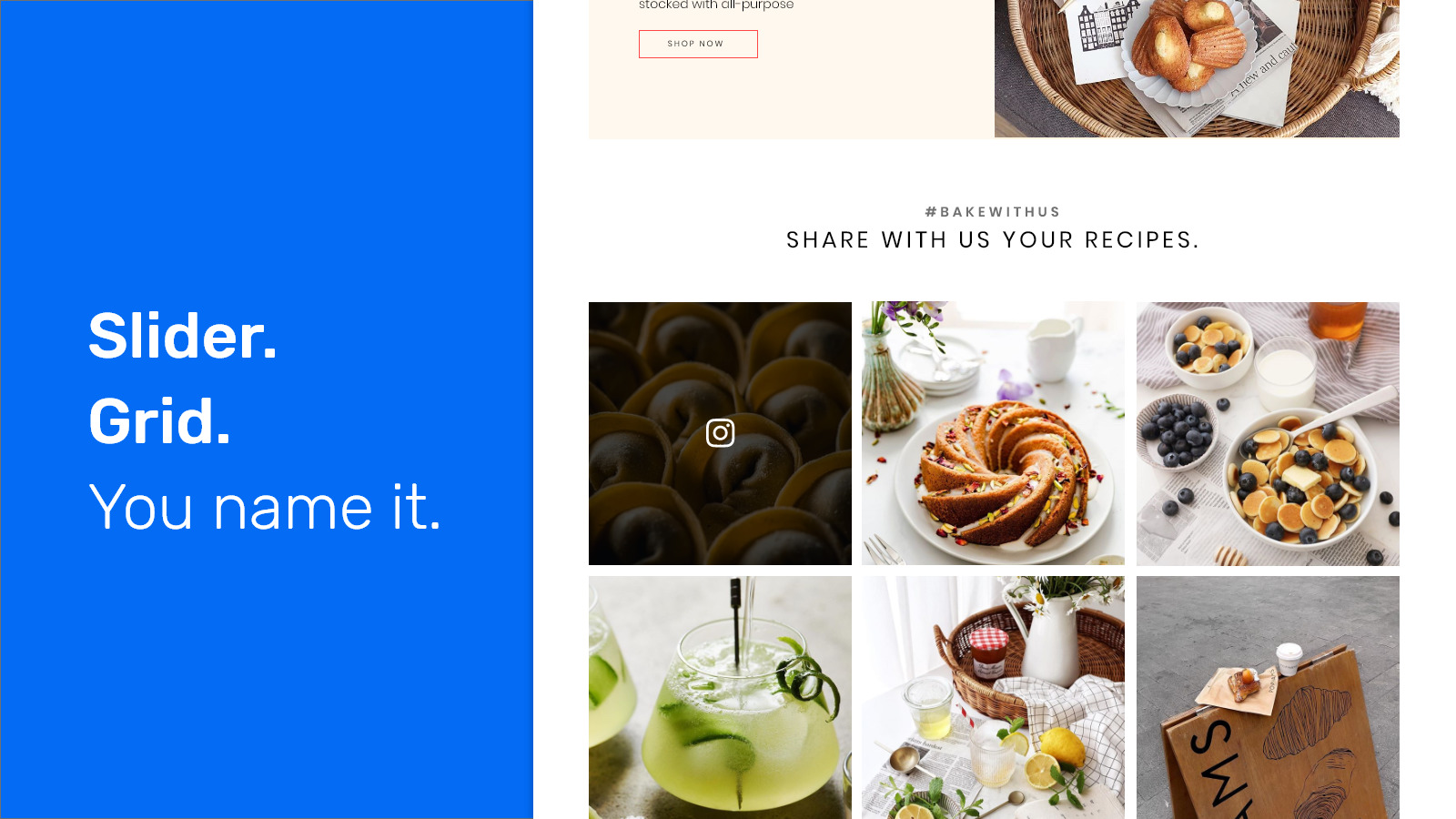The image appears to be an advertisement designed for Instagram, promoting a baking-related campaign. At the top, bold text reads "Stopped with Purpose," followed by a prominent "Shop Now" button. Below this, there is an inviting basket filled with assorted pastries. Beneath the basket, the text "Bake with Us" and the hashtag "#BakeWithUs" encourage viewers to join the baking community, share their recipes, and engage with the brand.

The lower section of the advertisement features six square images in a grid format, each showcasing a different baking-related item or scene:

1. The first image is an Instagram post that appears slightly darkened, featuring a pastry filled with chocolate cream.
2. The second image shows a spiral-shaped bundt cake adorned with nuts, presented on a pristine white plate. The background is predominantly white, with a hint of greenery from a plant in a vase.
3. The third image contains a bowl of fresh blueberries.
4. The fourth image depicts a large bowl filled with blueberries and orange slices, accompanied by a glass of milk.
5. The fifth image is of a refreshing beverage, potentially limeade or margaritas, garnished with lime slices.
6. The sixth image shows a bag set up as if ready for takeaway, hinting at convenience and on-the-go options.

The overall aesthetic is clean and appealing, designed to attract those with a passion for baking and culinary creativity.